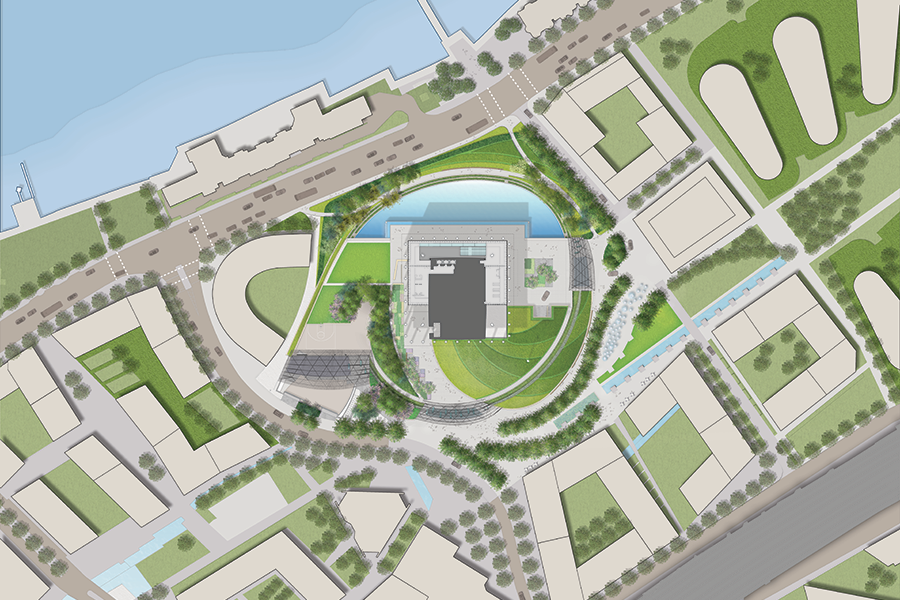The image portrays a detailed architectural drawing of an outdoor area, possibly a business complex or city park. Rendered from a bird's eye view, the map-like illustration features a blue section at the top left, likely representing a bay with docks. The complex is bordered by major roadways, depicted in the bottom right and along its edges, complete with symbols for cars. The central focus is a multi-story building distinguished by a swirling pattern and a semi-circular reflecting pond at its front. Surrounding this main building are various fields and green spaces, indicated by green areas symbolizing grassy fields and bushes. Numerous tan sections represent concrete walkways or sidewalks, and there are additional buildings of varying shapes, including U-shaped, oblong, and circular structures with courtyards. The complex is intricately connected by walkways and possibly a track encircling the central building, signifying a thoughtfully designed area from an elevated perspective, highlighting its functional and aesthetic characteristics.